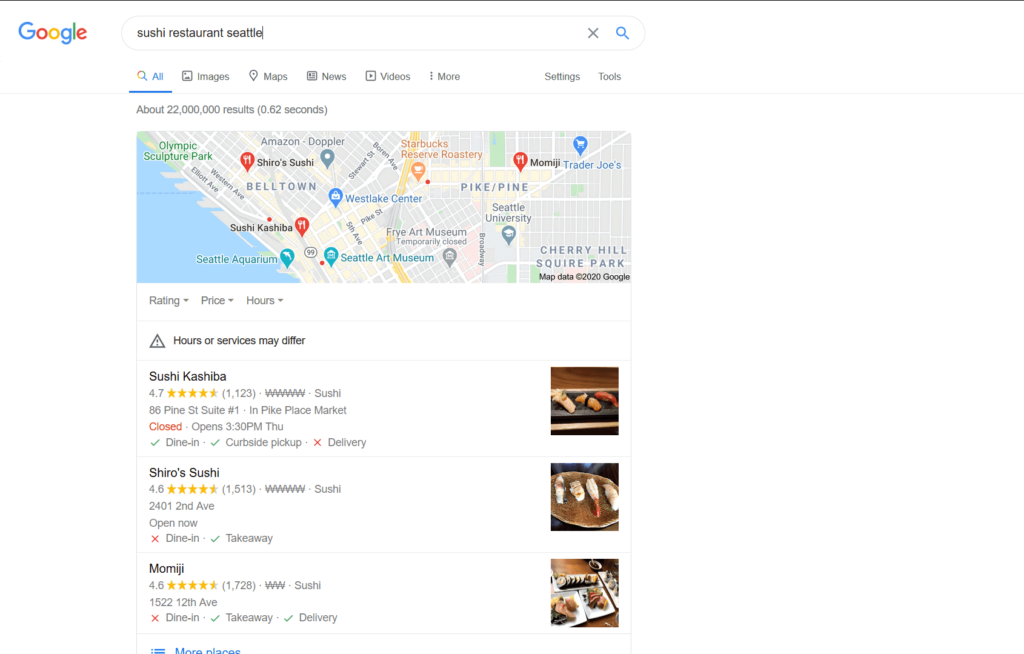This color photograph showcases a computer or notebook screen displaying a Google Maps search page for "Sushi Restaurant Seattle." At the top of the page, there's a header with options like All, Images, Maps, News, Video, and More, alongside buttons for Settings and Tools. Directly below, the page features a partial map of downtown Seattle marked with vertical red teardrop icons indicating the locations of various sushi restaurants—two on the left-hand side and one on the right.

Beneath the map, there's a section labeled with Rating, Price, and Hours, accompanied by a black-lettered warning inside a triangle symbol that reads "Hours or Services May Differ." Below this warning, three specific sushi restaurants are listed: Sushi Kabashi, Tsuro Sushi, and Mojin. Each listing includes star ratings, open or closed status, and exact locations. To the right of these details are three small images depicting dishes served at the restaurants.